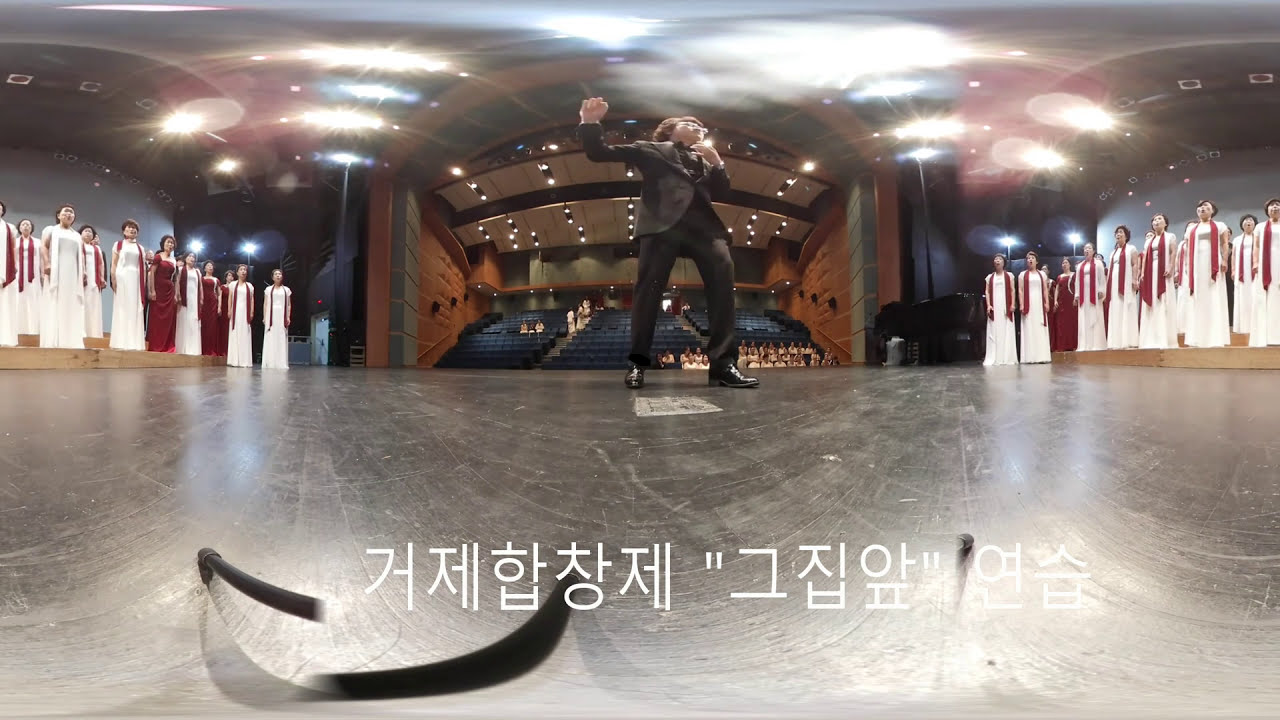In this detailed indoor theater scene, a central Asian man stands on a black stage, wearing a sharply tailored black suit, coat, pants, and shoes. His face is turned to the right with his left hand near his chin and his right hand raised, reflecting a poised, expressive gesture that suggests he might be performing. The camera lens distortion gives the image a unique beveled effect, warping the shapes around him but not diminishing the intensity of the moment. The stage floor, a scratched-up black surface, extends to meet a backdrop of wooden and gray-toned walls, above which strings of bright white lights and some blue-tinted lights illuminate the scene.

On either side of the performer, choir members stand elegantly in white dresses with red scarves draped over their chests, enhancing the visual contrast. Notably, two choir members on the left wear solid red dresses. The seating behind the man is empty, showcasing white seats arranged in stadium fashion, with some people visible in the lower right-hand section of the stands. Across the bottom of the image, white characters of an unfamiliar foreign language are printed, adding an enigmatic touch. The combination of colors—dominated by black, white, and red, with touches of blue and gray—enhances the dramatic atmosphere of this engaging stage presentation.